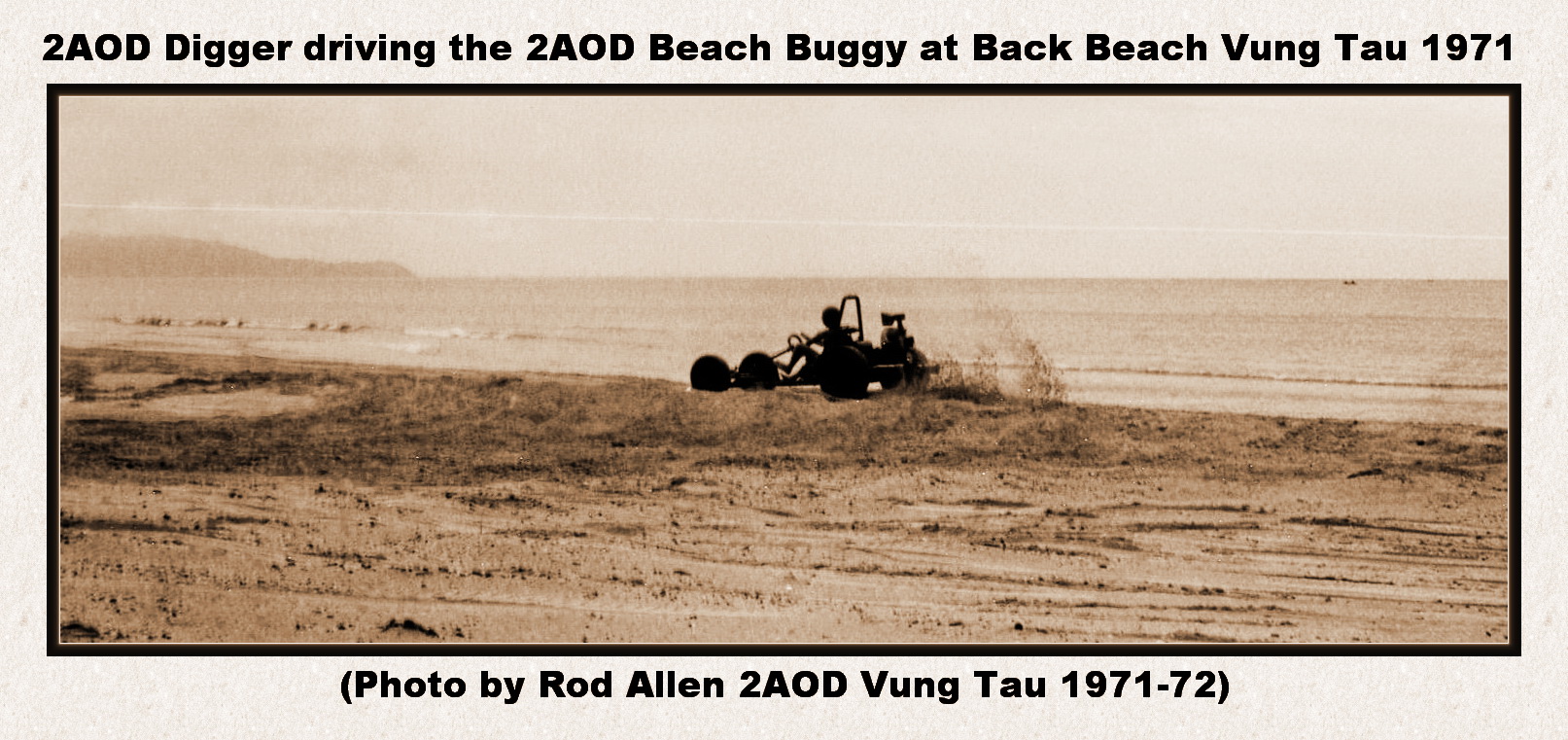This black-and-white photograph, subtly sepia-toned, captures a small dune buggy driving along the sandy edge of a beach, with muted brown hues dominating the scene. The photograph is oblong, nestled within a black line border on a gray background, and features sans-serif text at the top and bottom providing context. The text at the top reads, "2AOD Digger driving the 2AOD Beach Buggy at Back Beach Vung Tha, 1971," and credits the photographer, Rod Allen, from 2AOD Vung Tha, 1971-1972, at the bottom. 

In the image, the dune buggy, depicted mainly in silhouette with distinct outlines, has two large rear wheels and two smaller front wheels. The driver is visible with hands on the steering wheel and one leg raised, as if stepping on the gas. Behind the buggy, sand is being kicked up, hinting at movement, while small waves gently lap at the shore in the background. On the horizon, the setting sun creates a gradient that lightens towards the bottom of the image, with a small hill and distant mountains visible. A boat can be seen far off over the water, adding to the tranquil yet dynamic scene.